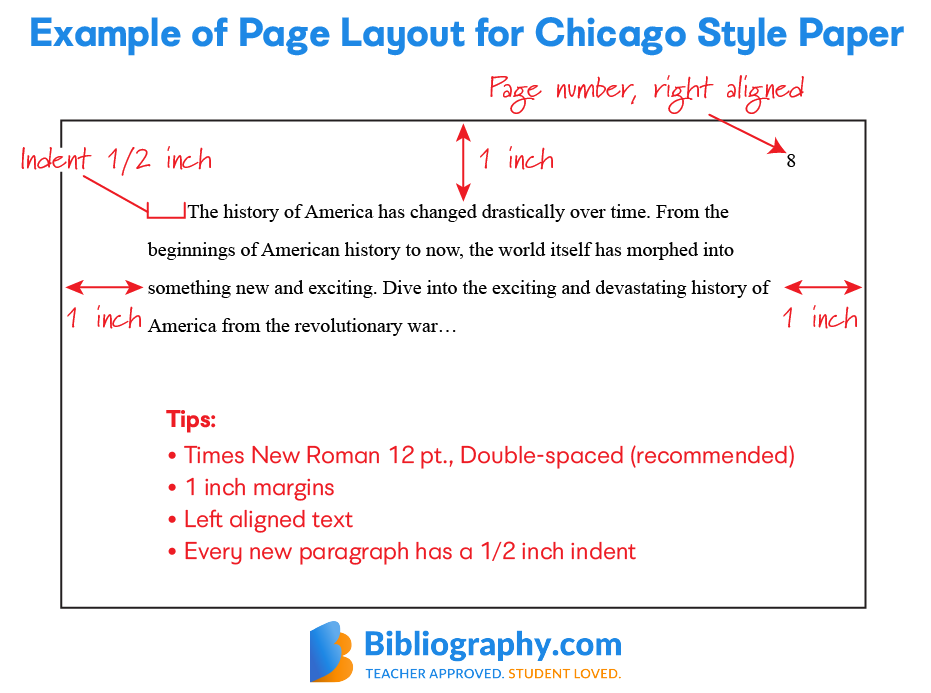The image is a detailed diagram illustrating the proper layout for a Chicago-style paper. At the top, the title in blue font reads, "Example of Page Layout for Chicago-Style Paper." The diagram features a paragraph of sample text which starts with, "The history of America has changed drastically over time. From the beginning of American history to now, the world itself has morphed into something new and exciting. Dive into the exciting and devastating history of America from the Revolutionary War..." Throughout the page, various elements are highlighted with red markers indicating formatting requirements: "page number, right-aligned," "one-inch margins," "half-inch indent for new paragraphs," "Times New Roman, 12-point, double-spaced recommended," and "left-aligned text." At the bottom in blue font, it features a logo and text reading "Bibliography.com," noted as "teacher approved" and in gold color, "student loved." The overall design includes a blue bee logo with an orange shadow, further emphasizing the site's branding.